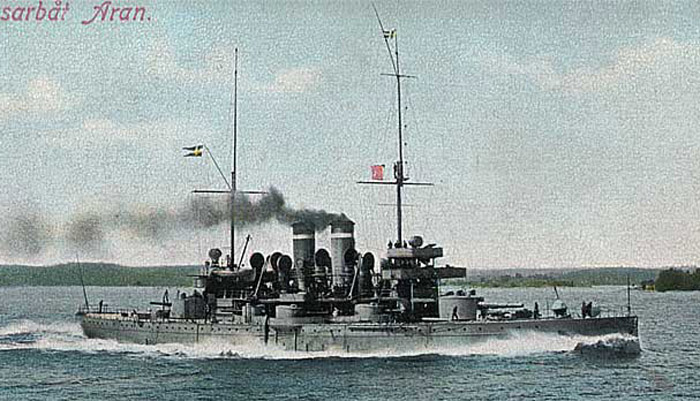This is a historical photograph, primarily in black and white but with some added colorization. The image captures a large World War I battleship in a bay, surrounded by verdant, jungle-covered hills that reach down to the water's edge. The battleship is constructed of gray metal and features two towering masts, each topped with flags. Two large smokestacks in the middle of the ship are belching out dark gray smoke, emphasizing the ship's active movement through the mysterious, bluish-tinted water. Small figures of crew members can be discerned on the deck. The sky shows slight blue hues, hinting at the colorization. At the top left corner of the image, the words "Sarbat Aran" are prominently displayed in red typeface, lending a postcard-like or archival quality to the photograph.